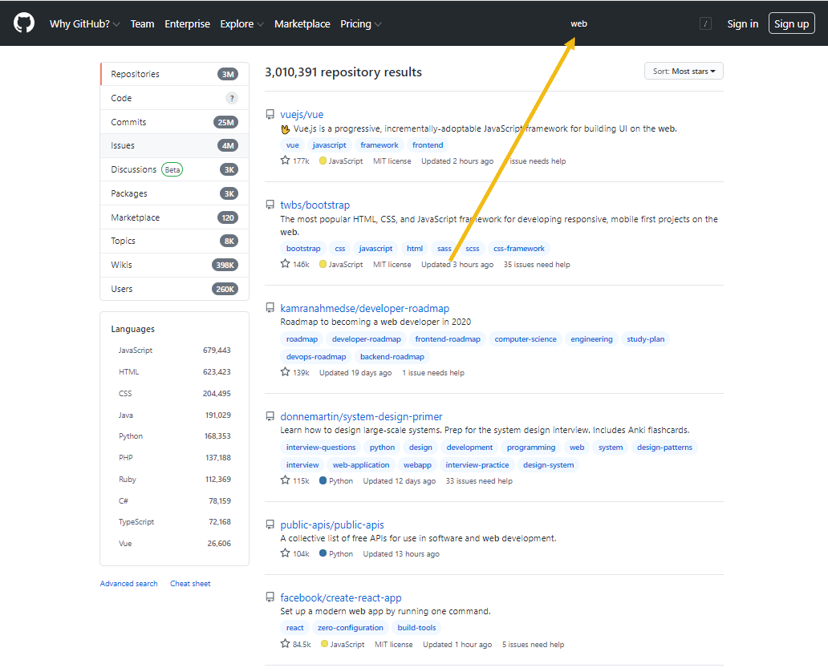This image is a screenshot of a GitHub webpage displayed with a small font and a slightly blurry resolution. The background color of the main body is white. At the top of the page, there is a black navigation bar spanning across the entire width. In the top right corner, the options 'Sign in' and 'Sign up' are present.

On the top left corner of the navigation bar, there is a white circle containing a cat silhouette icon, GitHub's logo. Next to it, in white text, are the navigation buttons labeled 'Why GitHub?', 'Team', 'Enterprise', 'Explore', 'Marketplace', and 'Pricing'.

Below the navigation bar, the left-hand side features a menu with various options: 'Repositories', 'Code', 'Issues', 'Discussions (beta)', 'Packages', 'Marketplace', 'Topics', and 'Wikis'. Following these, there are user-centric categories and a list of programming languages, including: 'Java', 'HTML', 'CSS', 'JavaScript', 'Python', 'PHP', 'Ruby', 'C++', 'TypeScript', and more.

In the main body of the page, at the top left, a bold text indicates "3,010,391 repository results." To the right, there is a sorting option available. Below, there are six repository results listed, each separated by a thin gray line. Each result features a blue headline with additional details underneath.

Annotations are present in the screenshot: a mustard yellow arrow has been drawn from the second result pointing up to the black navigation bar at the top. Additionally, the word "web" has been typed in black closer to the arrow's tip.